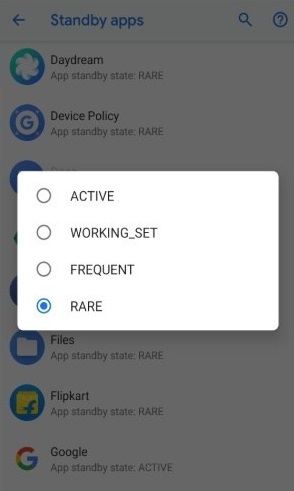This mobile screenshot displays an interface with a grayed-out yet fully legible background. At the top-left corner, there's a back button accompanied by the text "Standby Apps" in a bluish font. To the right, there is a magnifying glass icon followed by a question mark icon.

Directly below, the word "Daydream" appears with a small whirlwind-like logo next to it. The app standby state for Daydream is indicated as "rare." Further down, there's a segment labeled "Device Policy," featuring a bluish circular vault icon with the standby state also marked as "rare."

Centrally situated on a white background are four options with corresponding radio buttons: "Active," "Working set," "Frequent," and "Rare." The "Rare" option, located at the bottom, is selected.

On the grayish background below this section, the text mentions standby states for individual apps:
- "Files" with a white folder icon marked as "rare."
- "Flipkart" with a yellow folder and an 'F' insignia marked as "rare."
- "Google," displayed with the iconic Google 'G,' marked as "active."

The interface is clean and structured, providing clear statuses for various apps' standby states through a mix of icons and text labels.